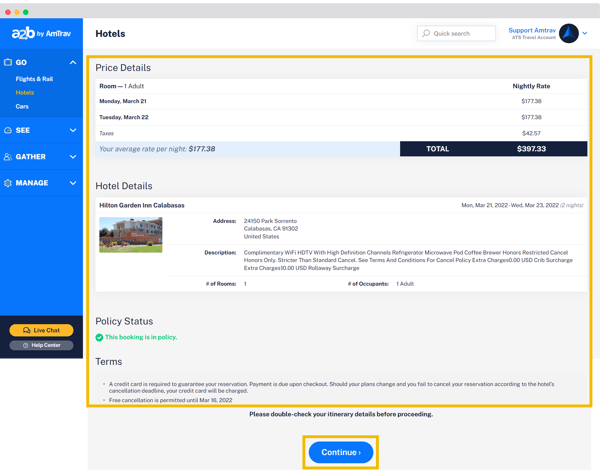Screenshot of a Travel Website Interface

This image appears to be a screenshot of a travel website. At the very top of the interface, there is a gray bar with red, yellow, and green dots on the left side, likely indicating window control buttons.

Along the left sidebar, which is in royal blue with white text, there is a logo that somewhat resembles a lowercase 'e', followed by 'z', 'b', all in lowercase, with the word 'Amitrav' (A-M-I-T-R-A-V) beneath it, although the text is slightly hard to read. Below this logo are navigation options including 'Go with flight and deals', 'Hotels' (highlighted in yellow), 'Cars', and then 'Hotels' again with a yellow context. Each of these options has a dropdown arrow, indicating further options.

Further down in the sidebar, there is a black background with two buttons: a yellow "Live Chat" button and a "Help Center" button.

The main screen features details about hotel bookings:
- In the upper left, it says 'Hotels', and the entire main content area has a yellow border to emphasize it.
- The section titled "Price Details" lists:
  - For one adult
  - Dates: Monday, March 21st to Tuesday, March 22nd.
  - Nightly rate on the far right: $177.30-something per night.
  - Taxes: $42.57.
  - Your average rate per night: $177.38.
  - Total amount: $397.33.

Below this are "Hotel Details" including:
- A thumbnail image of the hotel.
- The hotel's address, a brief description, the number of rooms available, and the number of occupants.

At the bottom of the section, there are additional options for policy status and terms.

In summary, this screenshot encompasses a travel booking interface with elaborate sections for navigation, price details, and specific hotel information, all presented in a user-friendly layout.